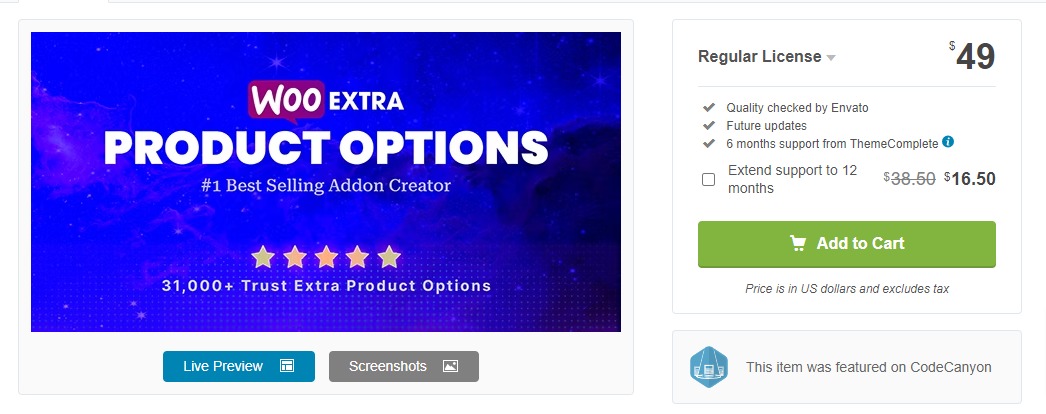The image likely portrays a screenshot of a webpage, although the absence of specific icons or interface elements makes it difficult to confirm the exact source. On the left side, a prominent blue box showcases an advertisement for "Woo Extra Product Options," labeled as the "#1 Best-Selling Add-On Creator." Directly beneath this, five stars are displayed alongside the claim, "31,000+ Trust Extra Product Options." The advertisement also offers clickable options labeled "Live Preview" and "Screenshots."

On the right side, the image details the pricing and support options for a "Regular License" costing $49, certified by Envato for quality. Additional mentions include future updates and a standard six-month support package from "ThemeComplete." There is a checkable box for extending support to 12 months, where the original price of $38.50 is struck through and replaced with a bold new price of $16.50. Adjacent to these details, a green box provides the option to "Add to Cart." Under this box, a note in italics clarifies that the price is in US dollars and excludes tax.

At the bottom of the advertisement, an icon's image is displayed with text beside it noting that "This item was featured on CodeCanyon."